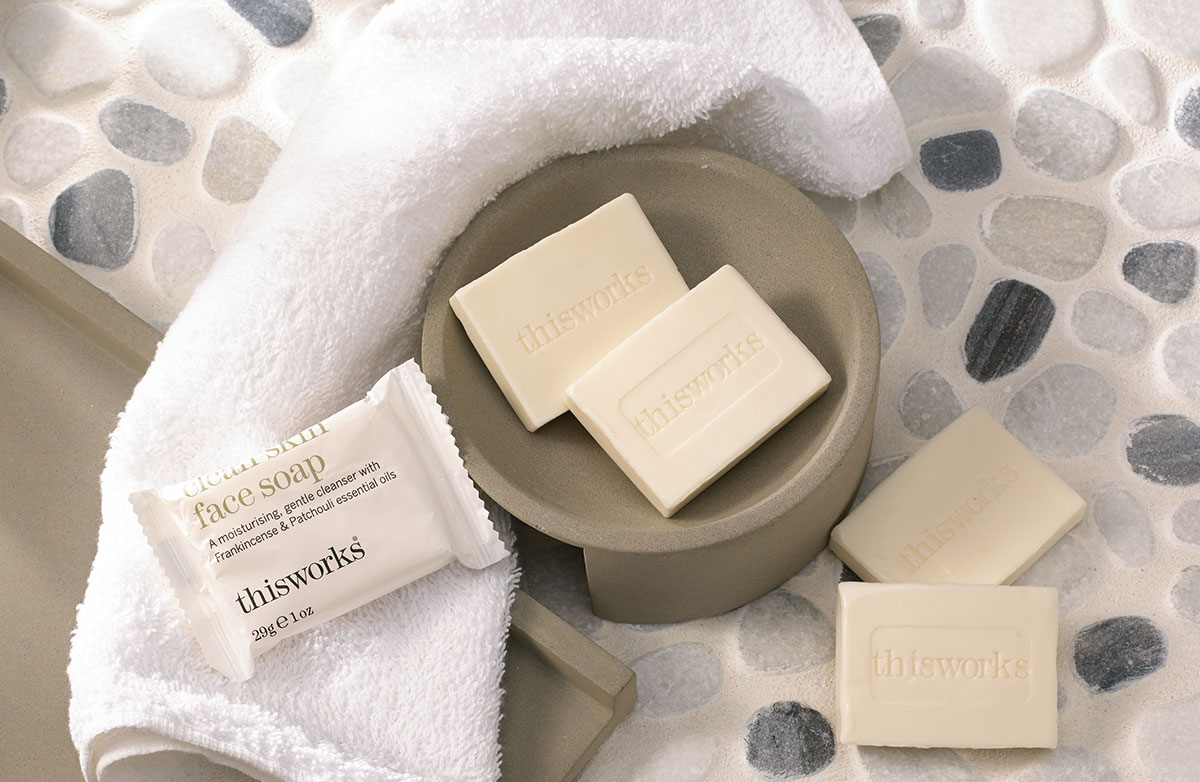The image depicts a countertop made of light and dark gray, irregularly-shaped stones with white grout. On the countertop sits a round, clay-colored or gray bowl containing two small, white, wrapped bars of soap that read "This Works." To the right of the bowl, there are two additional wrapped soaps, also labeled "This Works." A white hand towel is draped around the left side of the bowl's base, adding a soft curve to the scene. On top of the towel, there's another wrapped bar of soap labeled "Face Soap: A Moisturizing Gentle Cleanser with Frankincense & Patchouli Essential Oils," featuring perforations on its edges. The soaps, all small and reminiscent of hotel amenities, and the cohesive arrangement against the textured countertop create a visually appealing scene.